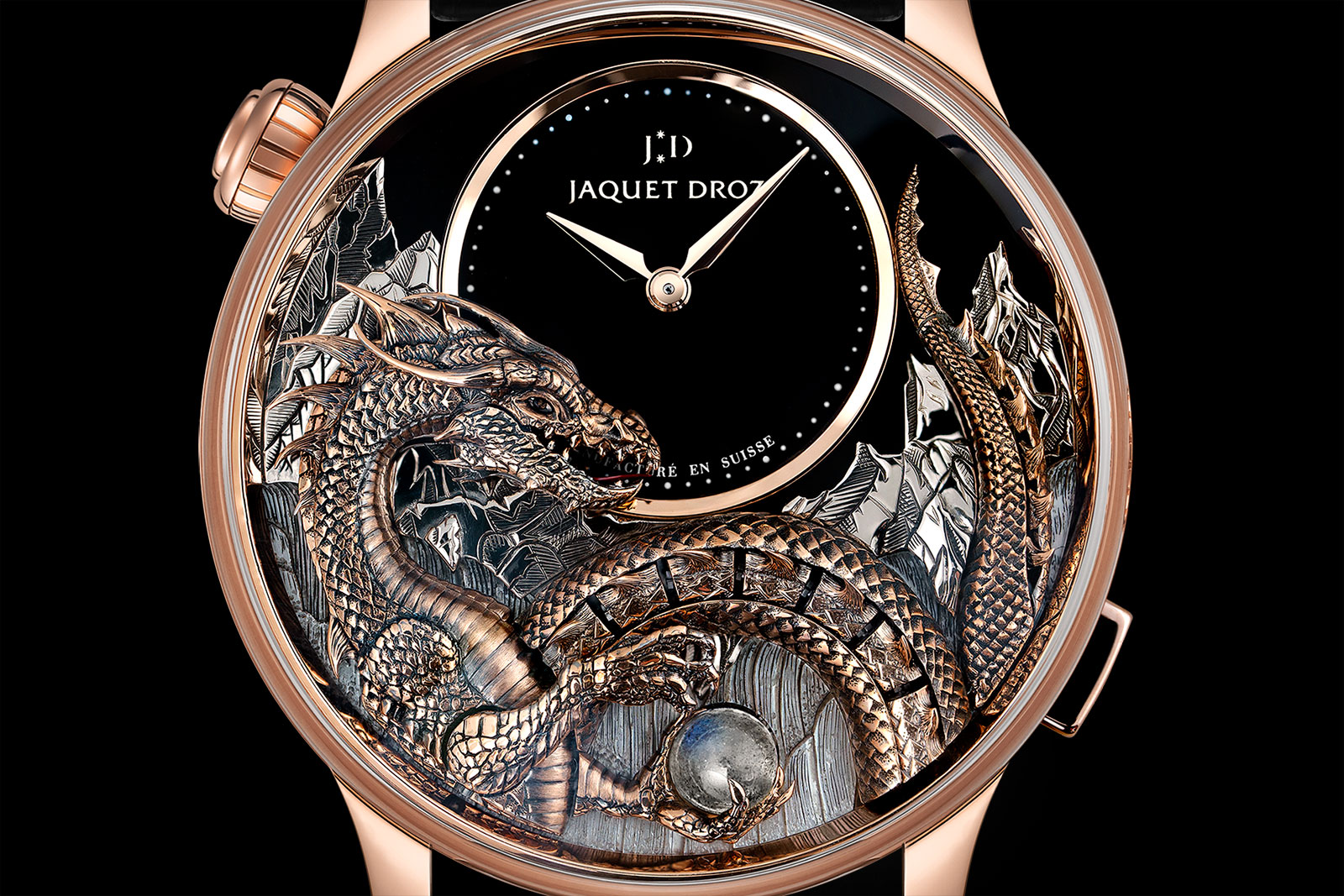This close-up photograph showcases an elaborate and luxurious wristwatch against a solid black background, which highlights the intricate details of the timepiece. The watch has a round face and is predominantly rose gold with a subtle contrast of copper and silver accents. The edges and face of the watch glisten with this rose gold hue, and at the top left, there is a winding knob.

Central to the watch's design is an exquisitely detailed dragon that appears at the bottom of the watch face. This dragon, crafted in metallic hues, features a long, curling tail and an open mouth. It holds a brilliant silver sphere or crystal ball in its claws, adding a touch of mystique to its design. The dragon's body and tail intricately wind around the watch face, creating an elegant visual flow.

The watch face itself contains a smaller, gold-toned circle where the time is shown, adorned with two gold hands set at about 10:10. There are no numerical markers, only sleek dots, emphasizing the minimalist design. Above the center of this circle, the initials "JD" are flanked by two stars, representing the logo of the renowned manufacturer, Jaquet Droz. The name "J-A-Q-U-E-T-D-R-O-Z" is inscribed in a refined font behind the hands of the watch, slightly obscured by the hour hand.

Additional details include metallic mountains subtly rendered in the background behind the dragon, adding depth and dimension. This watch, with its intricate craftsmanship and luxurious appearance, is a testament to high-end horological design, making it both a practical timepiece and a piece of art.